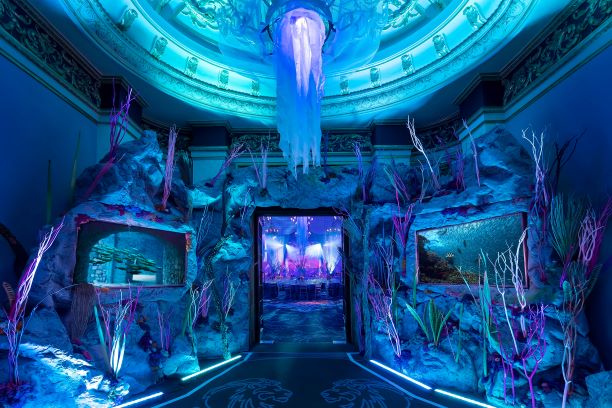This image appears to be a meticulously crafted, computer-generated interior of an artfully designed aquarium exhibit that predominantly utilizes a blue color scheme. Central to the image is an open doorway that gives a glimpse into another room, hinting at more marine displays beyond. Flanking this doorway are two large aquariums set into the walls; the one on the left is filled with green plants, while the right-side aquarium houses several small fish and various aquatic plants. The background features a water scene, possibly a digital rendering, that creates an immersive underwater ambiance.

Surrounding these elements are built-up rocky surfaces and coral structures, adding to the authenticity of the underwater theme. The ceiling, grand and expansive, is adorned with a striking chandelier that resembles cascading icicles or jellyfish tentacles, further enhancing the ethereal underwater feel with what looks like dripping or falling ice. This elaborate light fixture adds a touch of ornate elegance to the scene, casting a soft, almost mysterious glow throughout the room. The overall atmosphere blends artistic design with marine life, creating an immersive, aquarium-like experience.